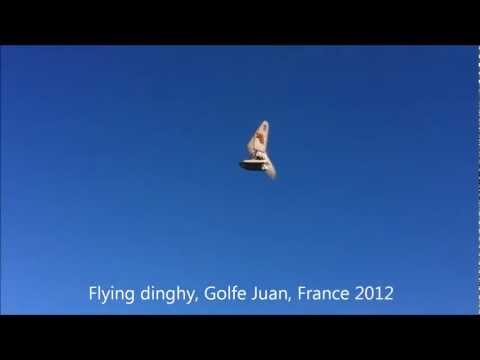The image features a serene, solid blue sky with an intriguing central object identified by the white text overlay as "Flying Dinghy, Golfe-Juan, France, 2012." This caption, prominently displayed near the bottom, is set in white font. The term "Flying Dinghy" suggests that the object, appearing to be a kite or balloon, is levitating in the air. The object itself, predominantly white with touches of red and black, contrasts starkly against the blue sky. Additionally, the image is framed by black borders on the top and bottom, reminiscent of a cinematic or theater mode presentation. The photograph's minimalist composition—with just the sky, the flying object, and the text—exudes a sense of calm and simplicity, capturing a unique moment from 2012 in Golfe-Juan, France.